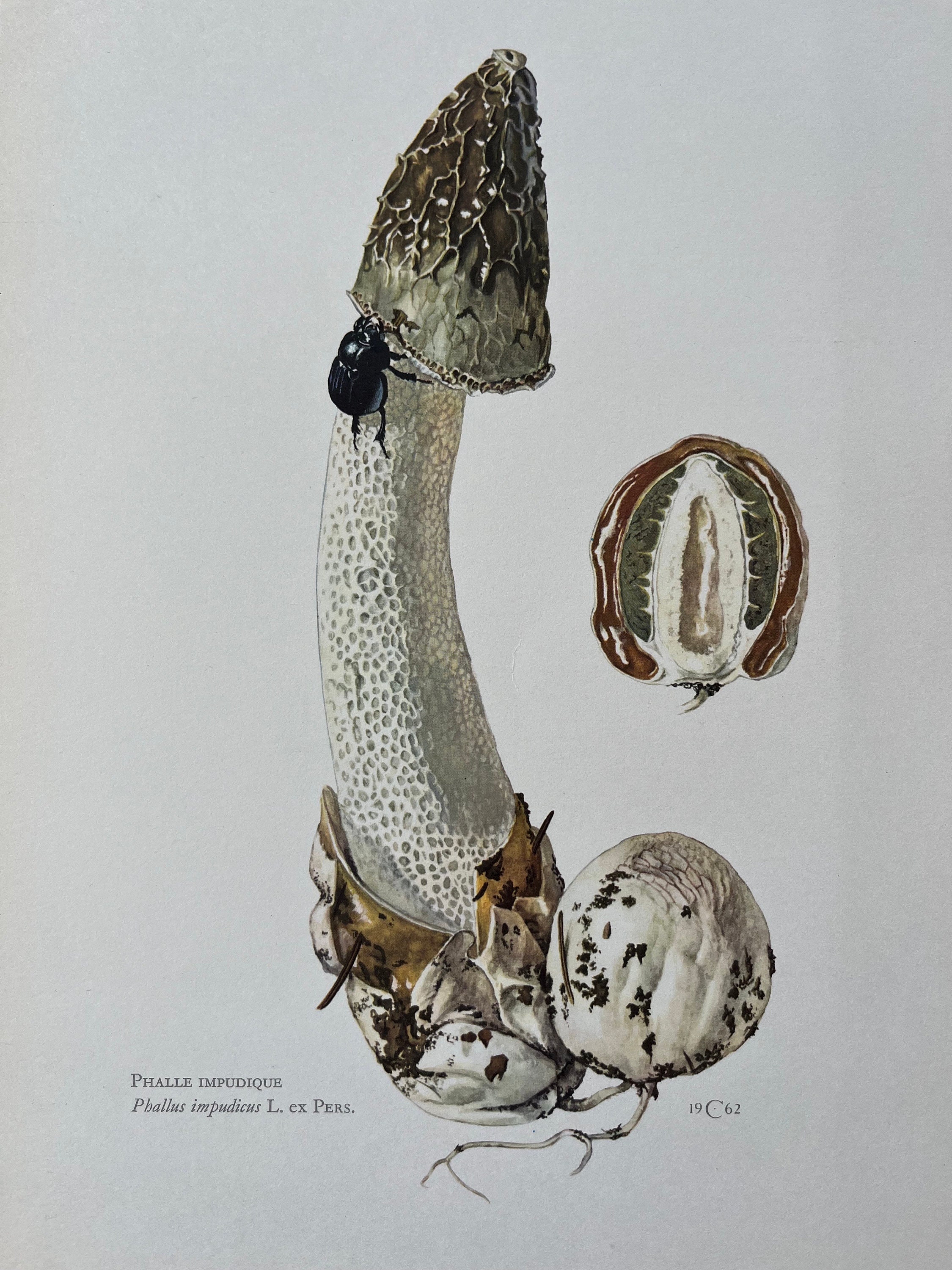This rectangular illustration features a naturally inspired, tall, and slightly curved white mushroom with a distinctly phallic appearance. The mushroom's stem has numerous porous dimples, reminiscent of Swiss cheese or sponge-like holes, and its surface appears textured and veiny. A black beetle is prominently crawling up the left side of the mushroom, making its way toward the conical, brown, and white cap. The base of the mushroom is engulfed in a mix of brown and white leaves, with two rounded bulbous areas, speckled with dirt, resembling testicles. To the left of the mushroom, there is a cross-section of a seed-like object featuring a brown exterior, a green lining, and a white core. The bottom left corner of the image contains text: "Phal. impudic." and "Phallus impudicus LX pers", while the bottom right corner displays "1962" with a "C." The entire scene is set against a white background.